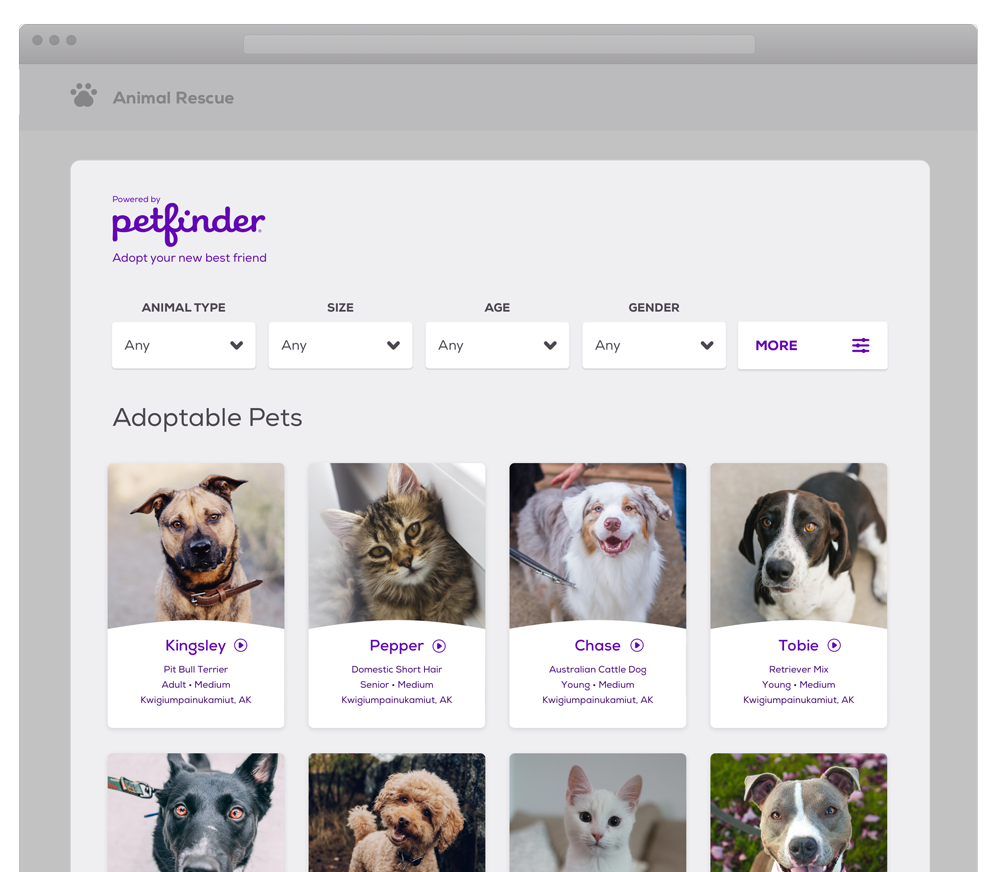This is a detailed screenshot of the "Animal Rescue" website powered by PetFinder, inviting potential adopters to "adopt your new best friend." The interface is designed with user-friendly features, including four comprehensive drop-down menus labeled "Animal Type," "Size," "Age," and "Gender." Each menu allows users to tailor their search by selecting specific criteria such as animal type (e.g., cat or dog), size (likely categorized by weight), age (either in months or years), and gender (male or female, with no further gender distinctions).

To the right of these menus is an option labeled "More" accompanied by radio buttons for additional filters, perhaps allowing users to refine their search by traits like fur type or hypoallergenic properties.

Below these menus, the section titled "Adoptable Pets" features a gallery of available animals:
1. **Kingsley** - An adult medium Pit Bull Terrier located in Quigley, Alaska.
2. **Pepper** - A senior medium domestic shorthair cat also residing in Quigley, Alaska.
3. **Chase** - A young medium Australian Cattle Dog, again from Quigley, Alaska.
4. **Toby** - A young medium retriever mix also available in Quigley, Alaska.

Additionally, the image hints at the existence of other adoptable animals, including three more dogs and a white cat, but their details are not fully visible as the image is truncated.